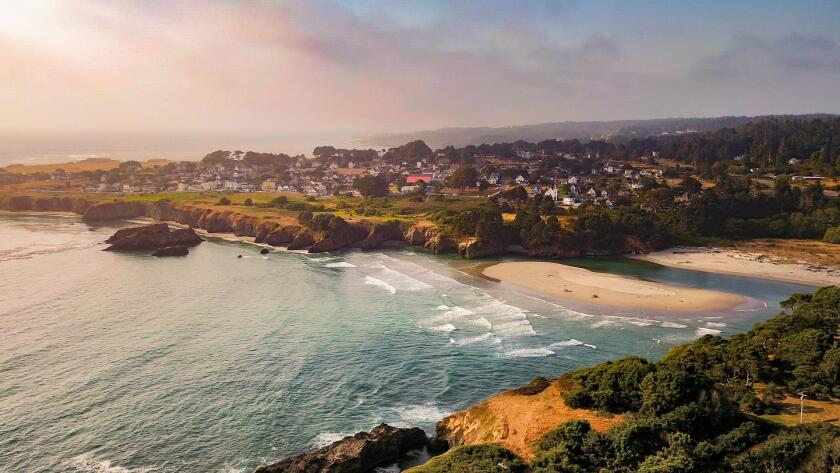This is a detailed photograph of a picturesque nature scene taken from a vantage point on a cliff, overlooking a serene and expansive bay. The foreground reveals some shrubbery and a telephone pole, emphasizing our elevated perspective. The water below is calm, with gentle waves lapping against a sandy beach area that surrounds a small water pool. Beyond this pool, the sandy beach continues and leads into a cove-like area with small strips of beach and cliffs topped with grassy stretches and scattered shrubs. To the left, the ocean meets the sand where some waves are softly crashing.

In the background, a quaint town is nestled along the coastline, characterized by numerous white houses and buildings. This village is ensconced in lush greenery and surrounded by a mixture of trees and undulating hills that gradually give way to a more mountainous area in the far distance. The sky above is a harmonious blend of pinkish blue and dusty blue hues, adorned with wispy clouds, creating the impression of a setting sun. The overall atmosphere is one of calm tranquility, with nature and human habitation coexisting harmoniously against the backdrop of a fading day.